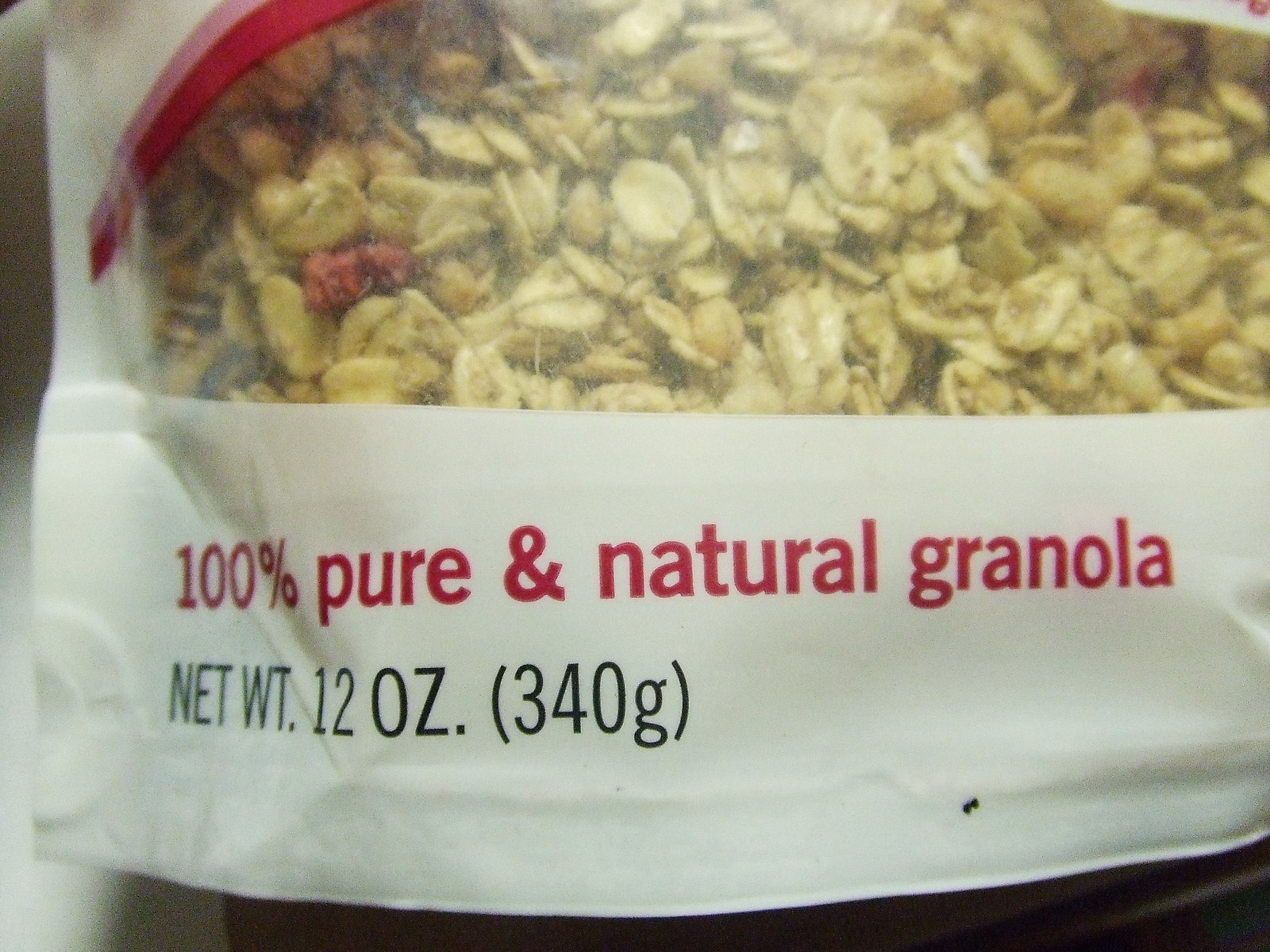This close-up photograph captures the bottom section of a bag of granola, focusing on the packaging details and the contents visible through a clear window. The bag is primarily white, with a bold red stripe and a softer pink stripe located just above the transparent section. Prominently displayed across the bottom in bright red text are the words "100% Pure and Natural Granola." Directly below that, in black text, the net weight is detailed: "Net WT 12 OZ (340g)." The clear window reveals a portion of the granola inside, showcasing a mix predominantly composed of light brown and tan oats. Interspersed among the oats are hints of red, potentially dried cranberries, and small, indistinguishable pieces that might be peanuts or other ingredients. The image cuts off the majority of the bag, emphasizing the granular texture and color variations within the granola, though not all contents can be clearly identified.